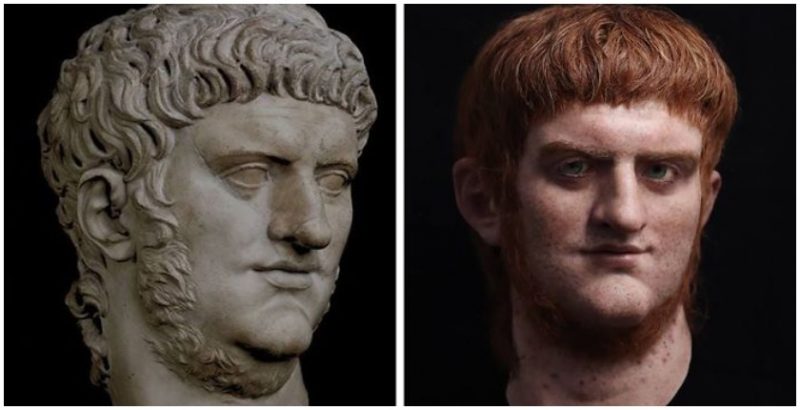The image features two side-by-side square photographs against a black background. The left photograph depicts a detailed sculpture of a head that resembles Roman Emperor Nero Claudius Caesar Augustus. The intricately crafted sculpture shows wavy, short hair and a beard that wraps around the bottom of the chin, extending into sideburns and around the neck. The head is slightly turned to the right, exposing the right ear and emphasizing the classical Roman features.

The right photograph is a colorized, photorealistic recreation of the same head, achieved through a combination of facial reconstruction, AI, and Photoshop. This artistic endeavor aims to represent how Emperor Nero might have appeared in real life. The recreated head shows red, shaggy hair that falls slightly over the forehead, staying above the eyebrows, and transitions seamlessly into sideburns and a full neck beard. The individual has a plump nose and green eyes, with a closed mouth, staring directly at the viewer. There are splotches on the neck, adding a lifelike texture, while the shoulders fade into darkness, creating a striking comparison to the original Roman sculpture on the left.